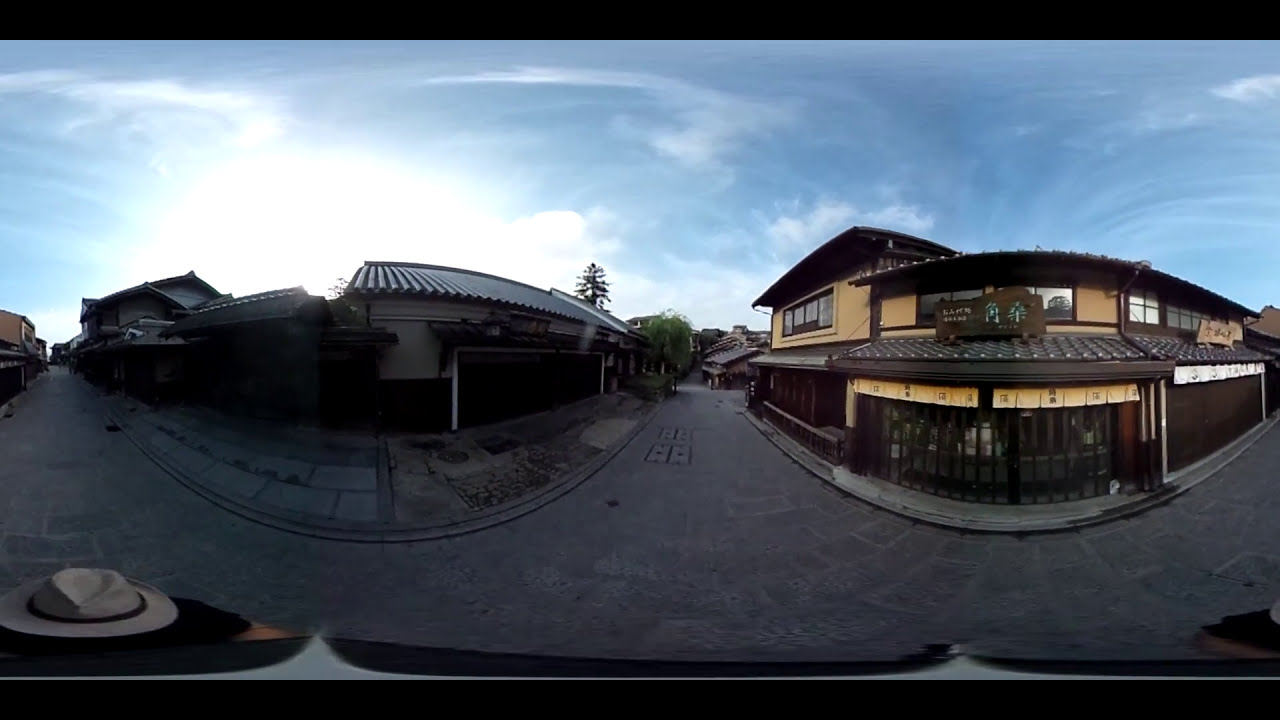The image captures a street view of an Asian town during the daytime, possibly early morning. The sky above is a bright, light blue adorned with misty white clouds, and the sun is shining from the left side, illuminating the scene. The photograph appears to have been taken from a fisheye lens which distorts the perspective, giving a curved appearance to the buildings and streets.

On the right side of the image, there is a yellow-colored storefront with large glass windows and a series of tan flags hanging above the entrance. Adjacent to this yellow building, there is another business featuring white banners and a closed rolling brown garage door. The rooftops of these buildings are rigid and steel-like, with a base that appears to be mahogany colored. 

The center street merges with the outside lanes, creating a sense of depth, lined with additional storefronts and trees visible in the distance. The buildings are predominantly tan and beige with brown tiled roofs. A prominent brown sign with light blue Chinese characters is visible on one of the beige buildings on the right. 

A person can be seen walking on the sidewalk, wearing a black short-sleeved t-shirt and a distinctive white fedora with a black brim, adding a touch of human presence to the tranquil street scene. The asphalt roadway and sidewalks of the streets suggest a well-paved, maintained urban area fenced in by various structures and further accented by the clear, blue sky overhead.